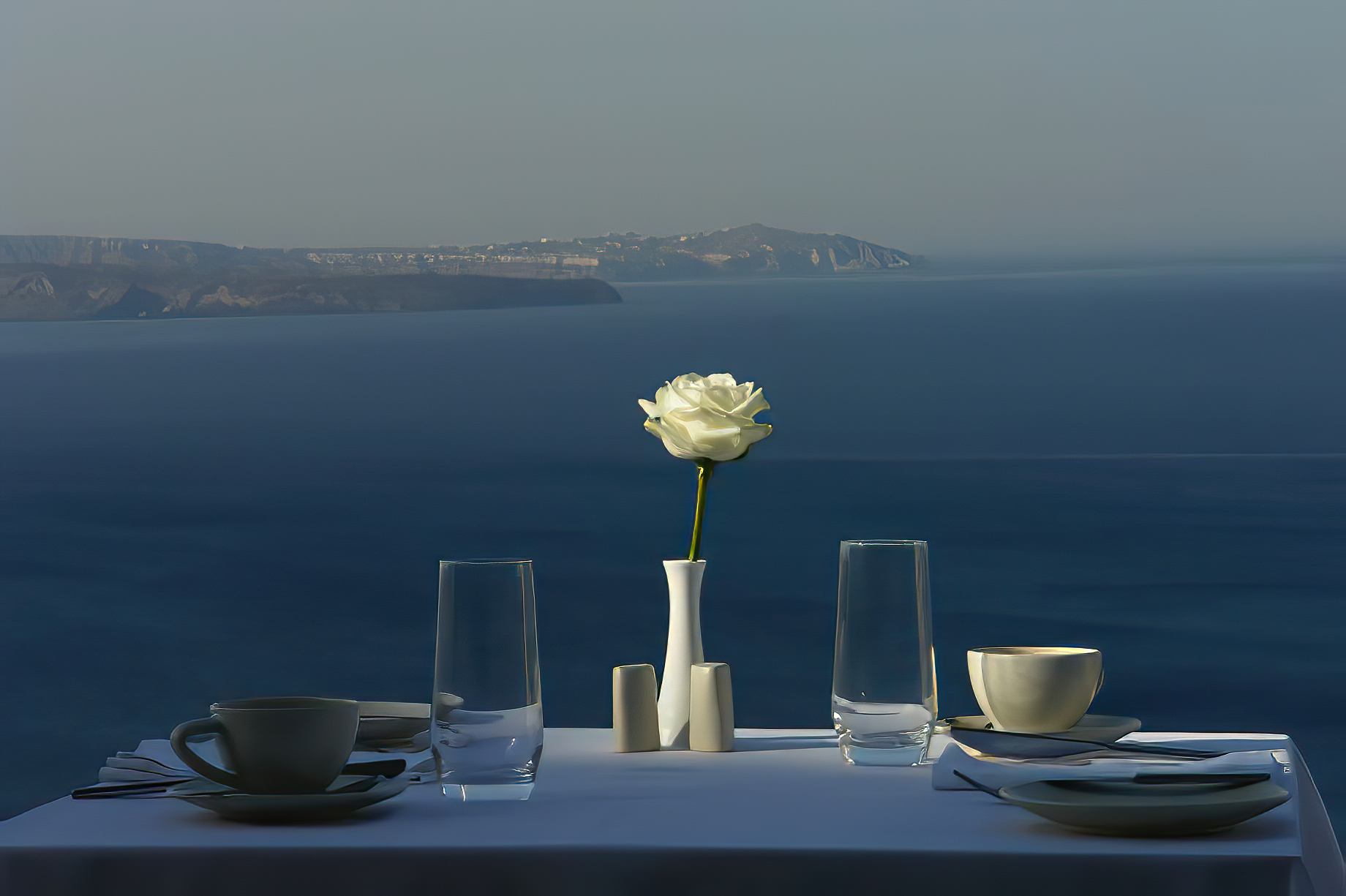This photograph captures a beautifully set table for two on an elevated deck or terrace overlooking a vast bay extending into the ocean. The rectangular table, draped in a pristine white cloth, takes center stage in the bottom portion of the image. Atop the table, place settings mirror each other on the right and left. Each setting includes a light brown bread plate, a napkin, and utensils, along with a semi-filled water glass and a small coffee or tea cup.

In the middle of the table, a small white vase holding a single cream-colored rose is accompanied by salt and pepper shakers. The rightmost edge of the table, basking in sunlight, contrasts with the more shadowed areas. 

The tranquil blue water of the bay dominates the vista beyond the table, framed by rolling brown and green hills that form two peninsulas. These landmasses stretch out into the water, one of which possibly features a row of houses. The distant horizon is capped by a sky in shades of grayish-blue, hinting at an overcast day. This serene and picturesque setting provides a calming backdrop to the intimate table arrangement.